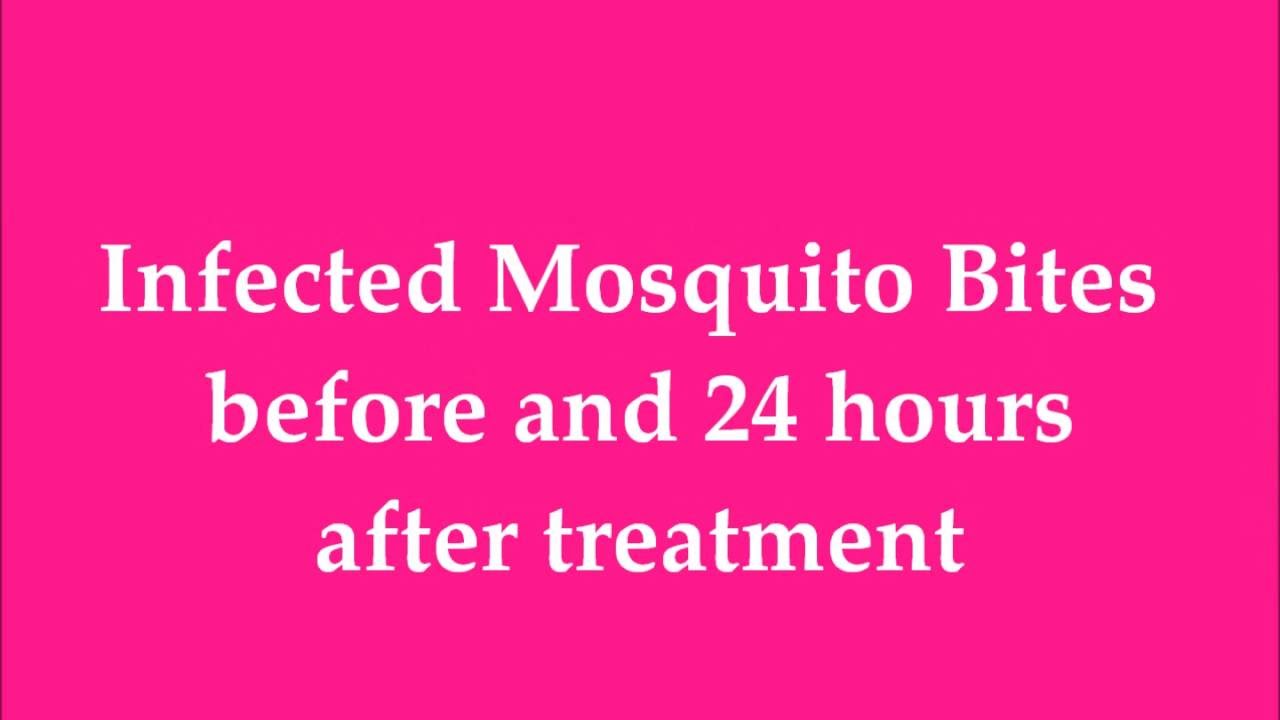The image features a bright, hot pink background that spans the entire frame, creating a vivid and attention-grabbing canvas. Centered within this backdrop is white text distributed across three lines, forming a pyramid-like arrangement. The top line reads "Infected Mosquito Bites," with each word capitalized. Directly below, the second line, written in lowercase, states "before and 24 hours." The bottom line, also in lowercase, concludes with "after treatment." This clean, text-only layout, devoid of any objects, appears to serve an informative purpose, likely for educational or digital presentation contexts, possibly preceding or accompanying comparative before-and-after images. The ample empty space above and below the text further emphasizes its centralized alignment and uncluttered design.